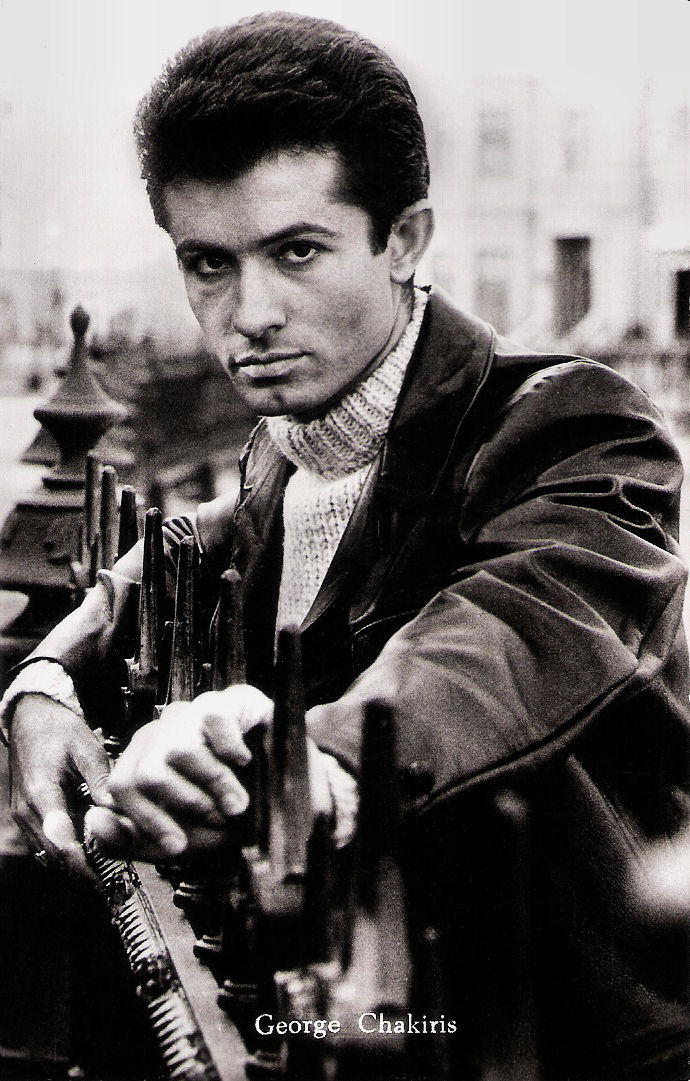This black and white photograph features a man named George Chakris, as indicated by the white text at the bottom center of the image. The man, clean-shaven with short, feathered-back black hair, stands against a pointed metal fence, his hands resting between the spikes. His body is angled towards the left side of the frame, though he gazes directly at the camera with an expressionless face. He is clad in a black leather jacket over a light-colored, knitted turtleneck sweater, with the cuffs of the sweater extending slightly past the sleeves of his jacket. The background reveals multi-storied townhouses with various square and rectangular windows, as well as a stairway leading up to a door. The further background details appear blurry, adding depth to the photograph. To the top left of the image, a more ornate section of the fence adds a decorative element, resembling a stylized turret.